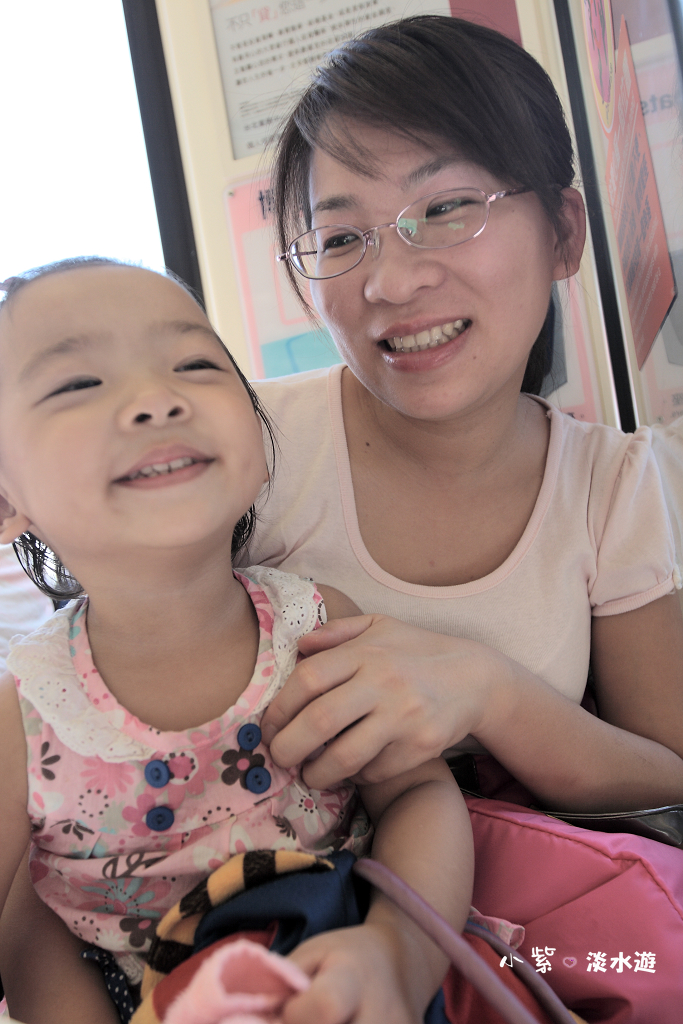The image depicts a smiling mother and her young daughter, both of Asian descent. The mother appears to be in her 30s or 40s, has blackish-brown hair, and wears glasses. She is dressed in a beige or light pink shirt and is looking fondly at her daughter. The young girl, aged between three to six years, has slicked-back black hair and wears a pink and white floral shirt. They are seated upright, possibly in an office, waiting room, or learning center. The background features artwork with Chinese or Japanese lettering, with additional text in the bottom right corner. Both mother and daughter exude happiness, captured in their shared smiles. The mother appears to be holding onto some bags, further adding to the candid feel of the photograph.